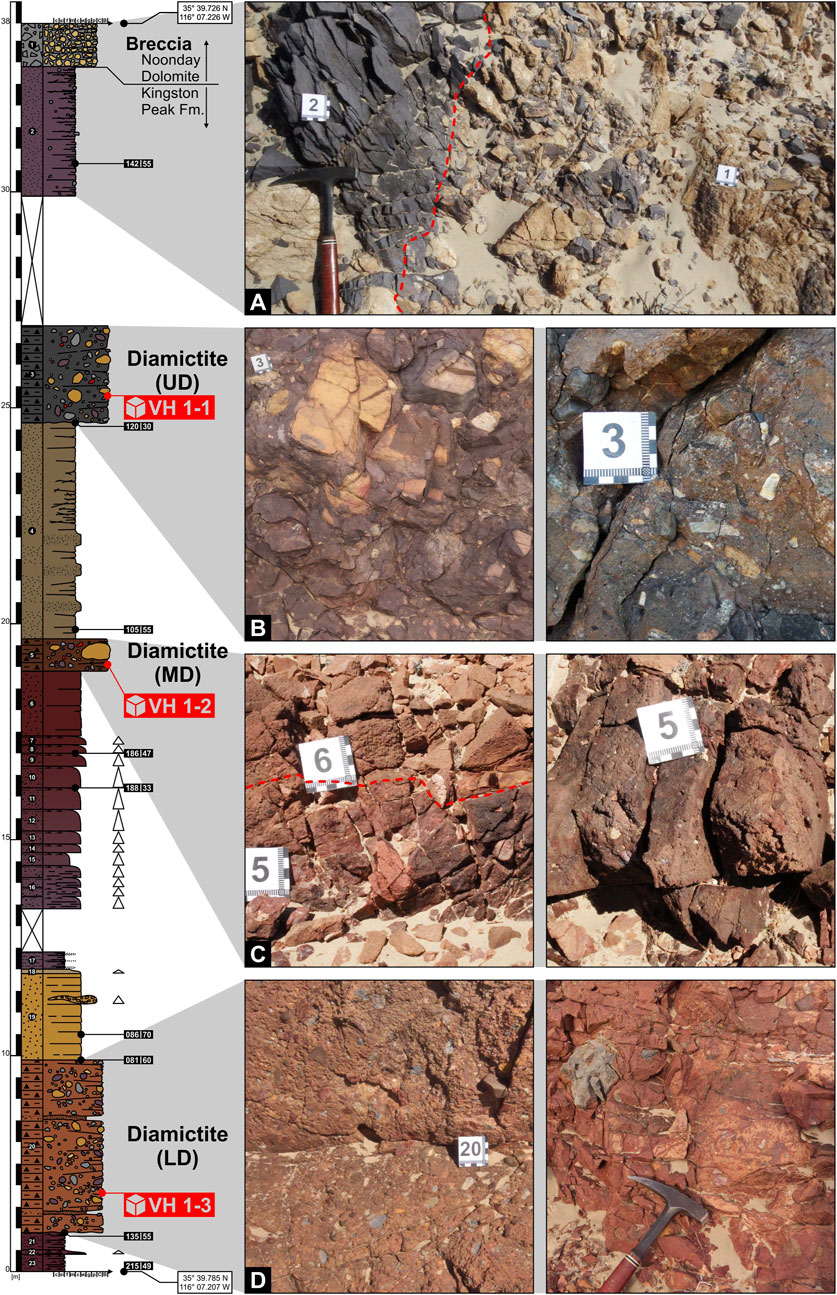The image displays a detailed geological study of various rock types, segmented into seven rectangular photographs. The larger photograph at the top showcases an extensive rock formation, possibly at an excavation site, featuring rocks labeled with geological terms such as 'Breccia,' 'Noonday,' 'Dolomite,' and 'Kingston Peak FM.' This image includes labels '1' and '2,' with a hammer-like instrument for scale. Below this, two rows, each containing two smaller rectangular photographs, depict different rock formations marked with the numbers '3,' '5,' and '6.' These rows are labeled 'Diamictite,' with additional descriptors 'MD,' 'UD,' and 'LD,' likely indicating specific types of diamictite. The final row also contains two smaller photographs, showcasing rocks labeled with '20' and another 'X.' The left side of the image features diagrams representing the geologic context of these rocks, indicating their positions within the Earth's stratigraphy. The rocks vary in color from brown and reddish hues to grayish tones, highlighting their diverse composition. Each section of the image is meticulously numbered for scientific classification and organization, providing a comprehensive overview of the types of rocks and their geological significance.